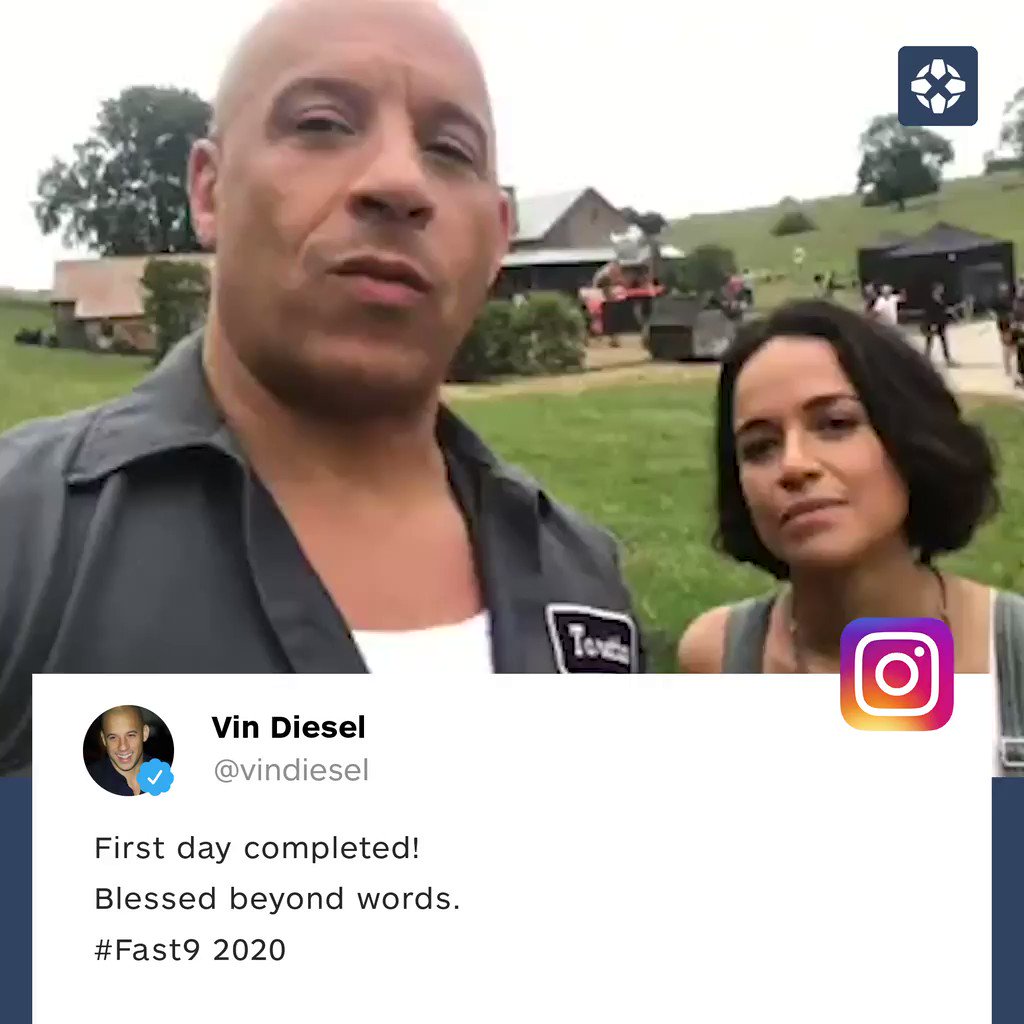The image is a detailed screenshot of an Instagram post made by Vin Diesel, featuring a picturesque outdoor setting. Vin Diesel stands prominently in the foreground next to Michelle Rodriguez. Both actors are looking directly at the camera with a backdrop of green grass, trees, and a clear sky, indicating a farmland or outdoor field location. In the lower part of the image, there's a white text box with black text. The Instagram logo is visible in the top right corner of this box, and on the left side, there is a small circular profile picture of Vin Diesel with a blue verification checkmark. Next to the profile picture, the name "Vin Diesel" is written with the handle "@vindiesel" below it. The text of the post reads, "First day completed. Blessed beyond words. #fast92020". The entire composition effectively captures the essence of a behind-the-scenes look at the filming of "Fast & Furious 9".